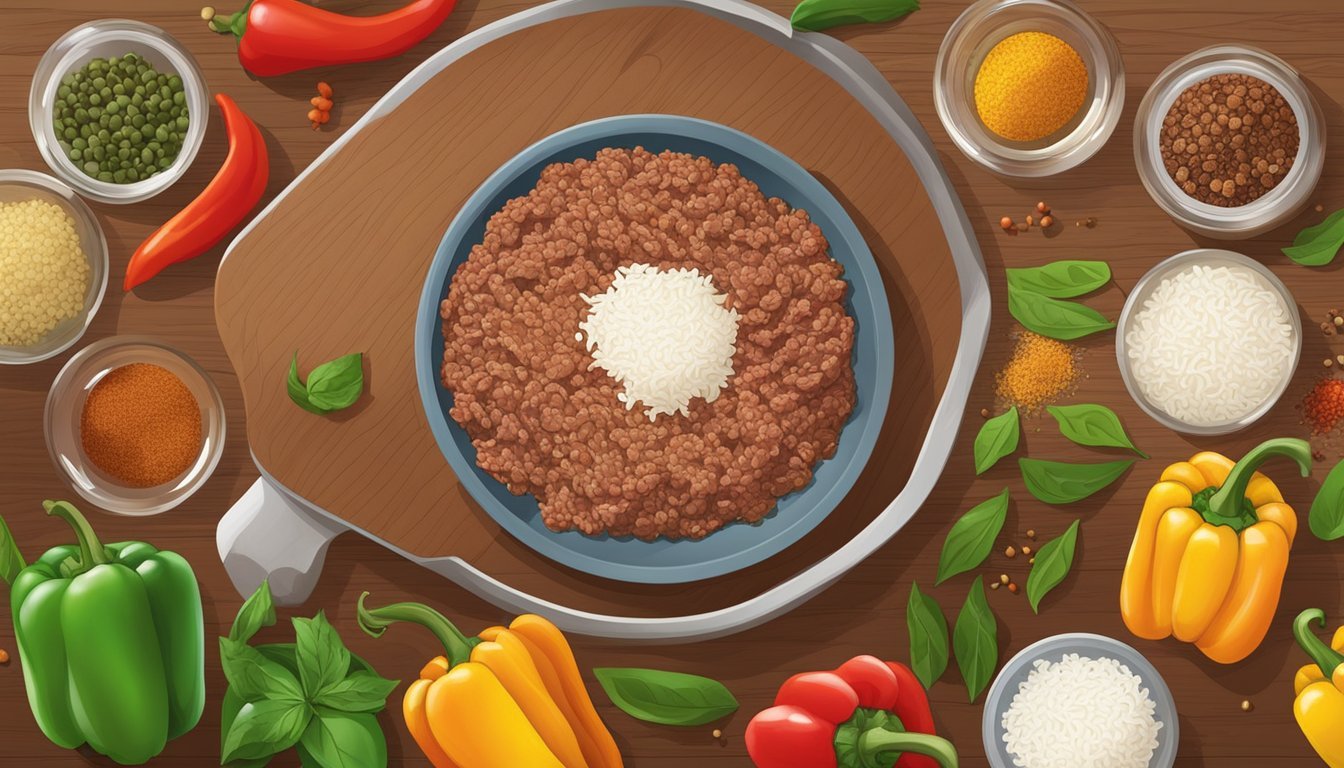This is a vivid cartoon-style artwork illustrating a food prep scene on a brown wooden tabletop. At the center of the table, there's a gray circular plate containing ground beef, which is topped with a small circle of rice. Adjacent to the plate, a single leaf is placed on the larger tray. Surrounding this central dish are numerous bowls filled with a variety of peppers — including a red chili pepper, green bell pepper, yellow bell pepper, and red bell pepper — alongside scattered basil leaves and hot red cayenne pepper. The bowls also contain ground spices, yellow powdery ingredients, white granulated substances, and lentils, all of which are neatly organized to be used in the dish. The vibrant colors of the food items, such as red, yellow, green, and white, enhance the artwork's visual appeal.